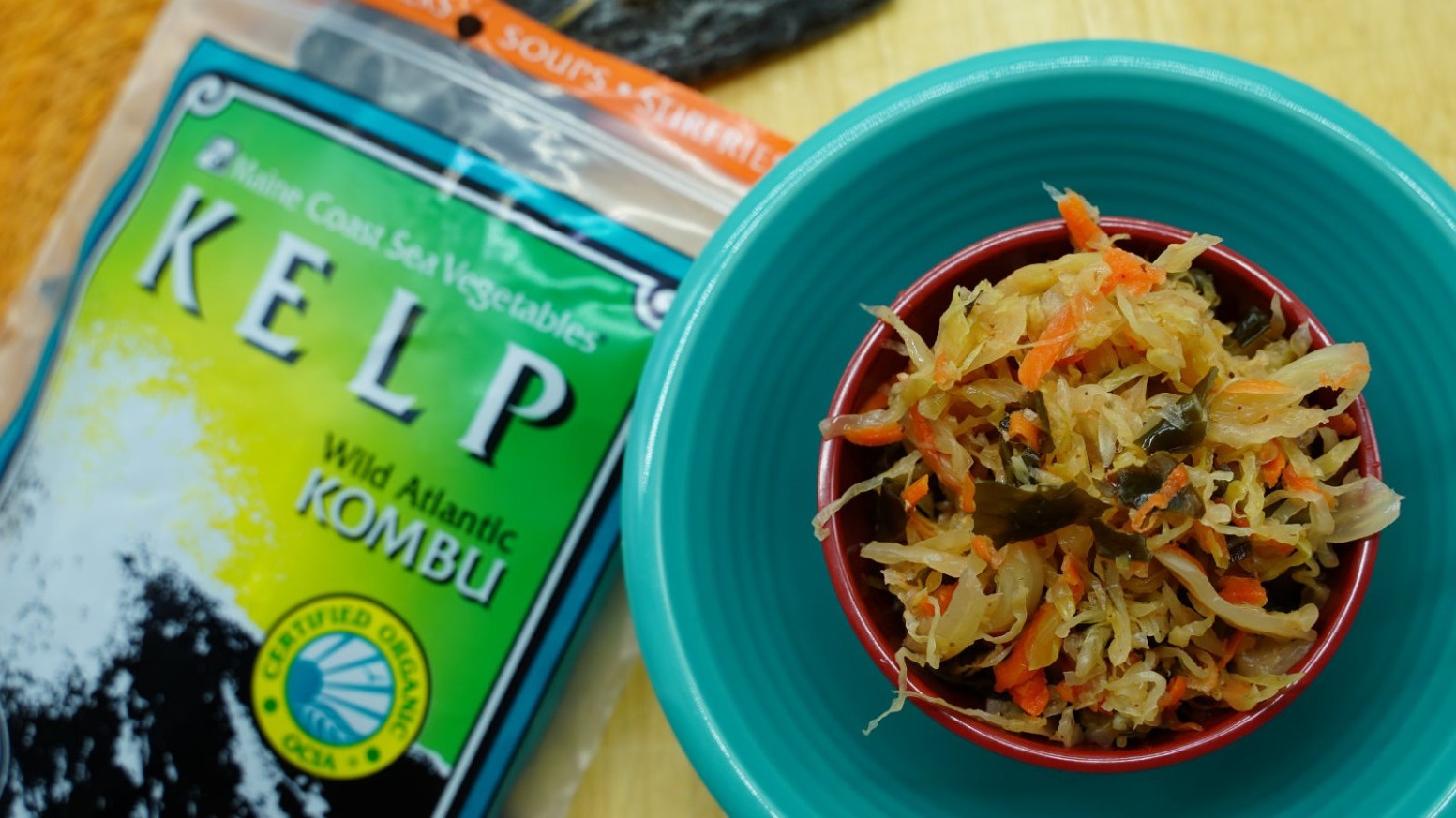This close-up image showcases a colorful, well-composed scene of a food dish and its ingredients. On the right side, there is a small red bowl filled with a mix of scalloped carrots, cabbage, and kelp. The red bowl is nested inside a larger blue bowl, both placed atop a turquoise plate. The dish has a stir-fried appearance, with the vegetables visibly coated and slightly glistening. On the left side of the photo, set against a light wooden table, is a clear plastic package of kelp. The package features a green and blue label with white lettering that reads, "Main Coast Sea Vegetables," followed by "KELP" and "Wild Atlantic KOMBU" in black and white. The top orange banner on the package highlights its suitability for soups and stir-fries. A circular emblem on the package marked "Certified Organic" is depicted above an image of waves crashing against a rocky shore, emphasizing the kelp's origins from the Atlantic coast of Maine.